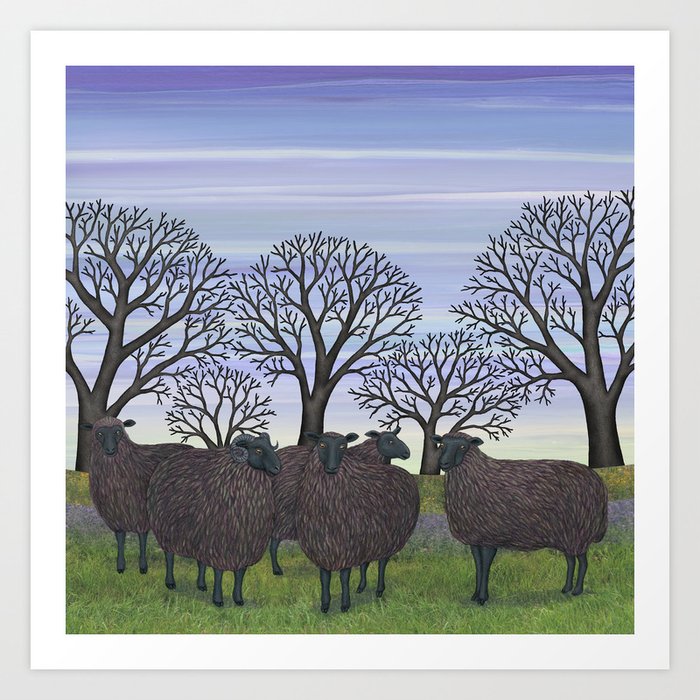The image depicts a detailed painting hanging on a white wall. The central focus is a square canvas featuring five black sheep, including one black ram distinguished by its spiral horns. The sheep are illustrated with fluffy black fur and black faces, standing amidst a grassy field in an outdoor setting. The grass is vividly green, with a small grey path separating two grassy areas. Surrounding the sheep in the background are five leafless, barren trees, each with multiple branches. The sky above them is artistically rendered with streaks of blues and whites to represent cloud cover, creating a semi-realistic and dynamic atmosphere. The entire scene is enclosed within a white border, accentuating the vivid colors and intricate details of the artwork.